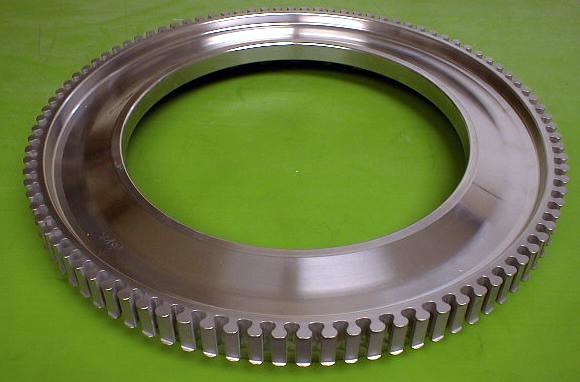A large metallic ring or cylinder, possibly from industrial machinery or a truck, is laying flat on a lime-green vinyl surface. The cylinder, made of silver or chrome, exhibits a shiny, gunmetal-gray hue with some white highlights likely caused by overhead lighting, suggesting the photo was taken indoors. The object features a central hole that provides a clear view of the green background. Along its ridges, evenly spaced rounded grooves resembling zipper teeth encircle the entire perimeter. The photo, taken from a close angle, hints at some faint markings or etchings at the bottom left of the cylinder, though their exact nature is indistinct. The unique design includes a slightly raised middle section that curves inward and upward, differing from the conventional gear structure.